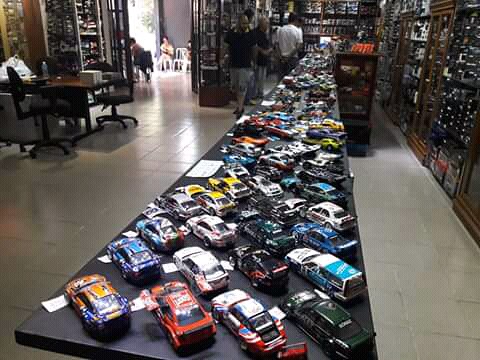The image depicts the interior of a shop resembling a hobby store, filled with a vast display of miniature and model cars. At the center of the store, there is a long black table, seemingly composed of multiple tables pushed together, showcasing an extensive collection of toy cars in various colors, sizes, and types, including casual cars and racing models. Each car is meticulously positioned with tags, and they all face towards the left of the image. The store features a tiled floor, lending it a clean and organized appearance.

Along the right side of the shop, there's a wall of dark wooden shelves filled with various objects, though the items on the shelves appear blurred and indistinguishable. To the left, there's a desk accompanied by two office chairs, creating a cozy, inviting spot. In the background, three people are visible; two men dressed in black and one person in white, seemingly browsing or shopping. Towards the image's top left corner, an open doorway reveals bright sunlight and people seated on white patio chairs outside, adding a dynamic contrast between the indoor and outdoor environments. Additionally, more display shelves line the left wall, further accentuating the shop's array of hobby items. The overall ambiance feels like a blend of a meticulous showroom and a casual gathering spot, perhaps giving off a library-like vibe due to its organized yet inviting setting.